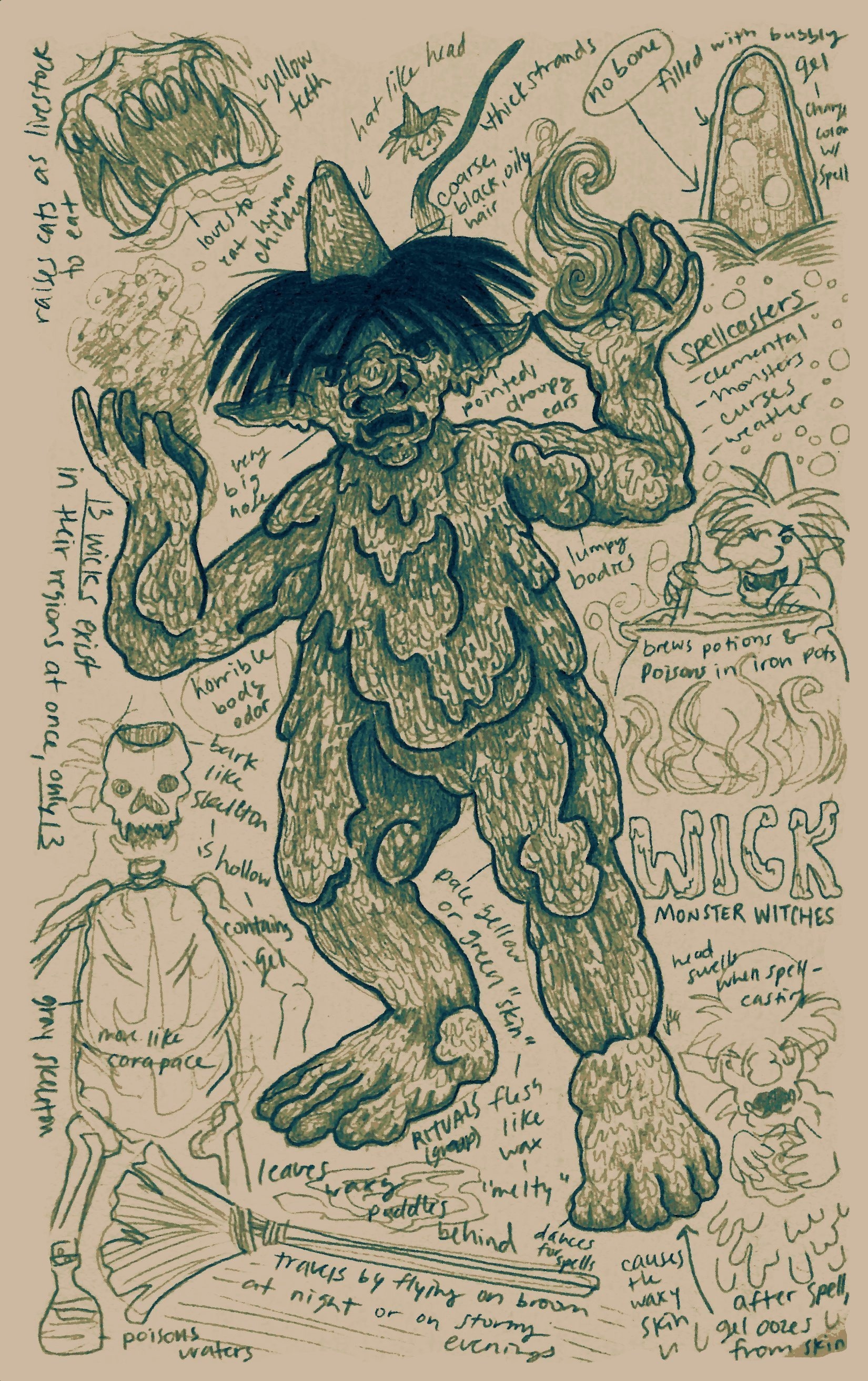This is a detailed poster set against a light brown, almost ochre background, with a striking central image of a grotesque ogre-like monster. The monster, reminiscent of a menacing straw man from "The Wizard of Oz," has an uncanny appearance with greenish skin, black, pointy hair, and an unsettling, fang-filled mouth poised as if to bite. His face is distorted, giving the impression of a half-melted wax figure capable of magic. Surrounding the central figure are various eerie sketches and writings in dark green, adding to the chaotic feel of the poster. Notably, phrases such as "No bone filled with my bubble gel," "I change your spell," and "Wick monster witches" are scrawled across it. Additionally, there's a skeletal figure perched in the lower right corner and a witch brewing potions in an iron cauldron on the right side, with a broomstick suggesting flight on stormy nights. The left lower corner ominously mentions "poisonous waters." Each element combines to create a vivid and eerie scene that tells the concept of a monstrous world filled with spellcasters and dark magic.